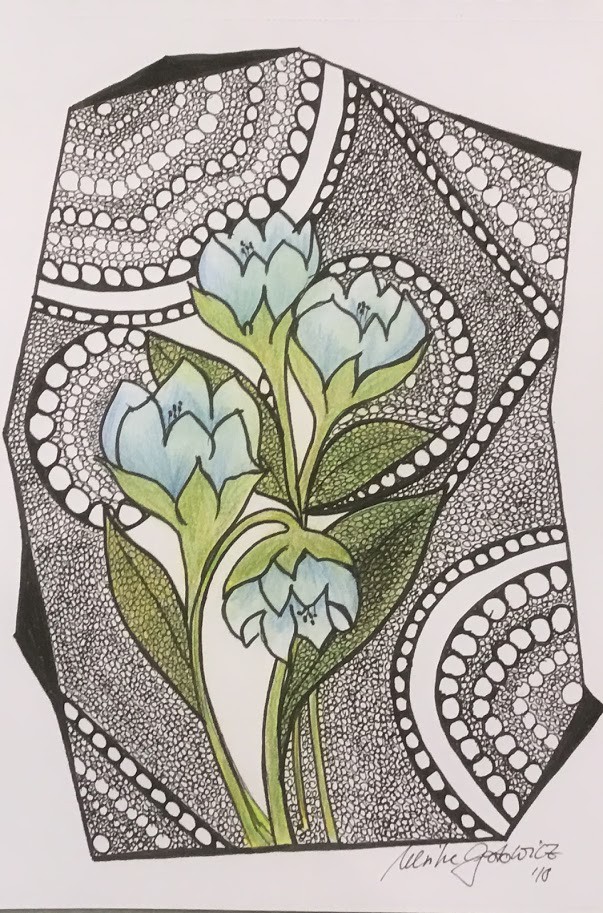This hand-drawn sketch, created using black marker or pen and shaded with colored pencil, features a vibrant centerpiece of four blue flowers with green stems and leaves. Surrounding the flowers is an intricately detailed circular pattern, characterized by a mesmerizing swirl of repeating lines and variously sized circles in black and white. The artwork is enclosed within an irregularly drawn black border that frames the composition. In the lower right-hand corner, the piece is signed with what appears to be the initials "M.G." and dated 2010, although the signature is somewhat unclear.